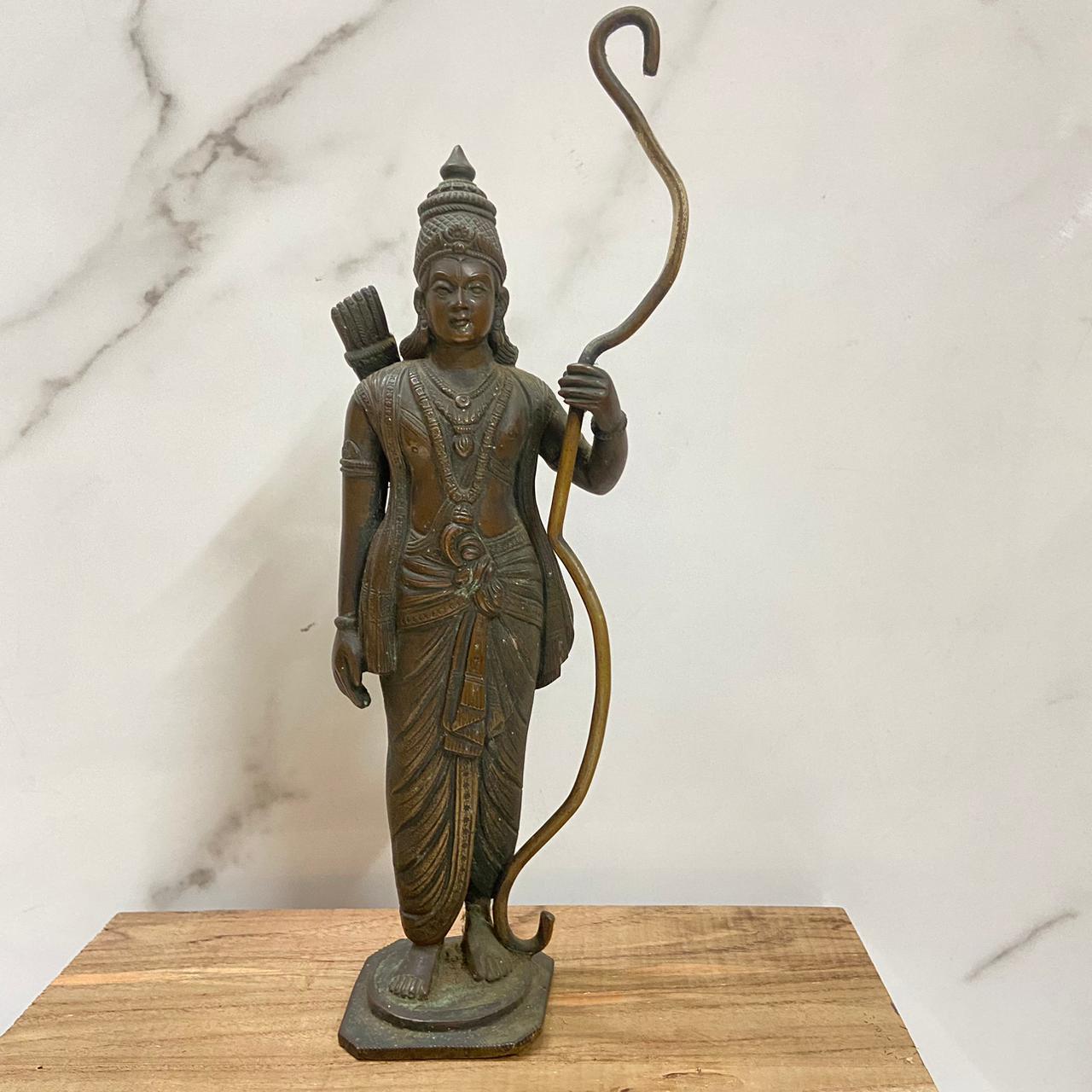The image features a bronze statue of an oriental or possibly Indian figure, characterized by a highly detailed and elaborate appearance. The statue stands barefoot on a square base with a rounded inner platform, placed on a small wooden surface that extends beyond the visible frame. The attire includes a long robe or sarong covering the bottom half and a vest-like top or tunic that's open to reveal the chest. A large belt cinches the waist. The figure's head is adorned with an elaborate, pointed headdress. 

In its left hand, the statue clutches a long, sinuous staff that intertwines from the foot up to the shoulder, ending in various hooks and curls – resembling a decorative shepherd's crook, though possibly intended to be a bow given the presence of arrows behind the back. Three layers of intricate necklaces drape around the neck, adding to the figure's ornate appearance. The background is a white marble wall with subtle gray streaks, providing a stark contrast to the dark, bronze hue of the statue.